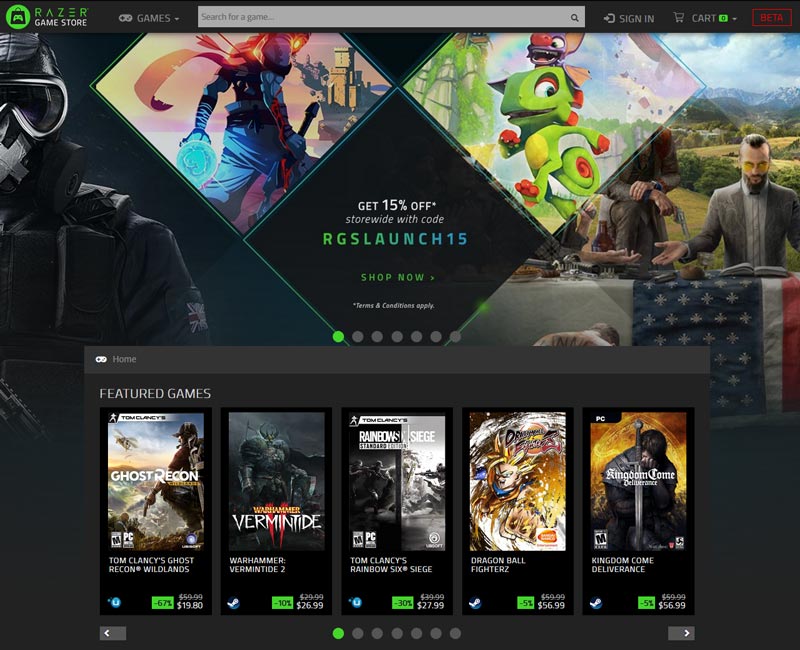In the top left corner of this image, the "Razer Game Store" logo is prominently displayed. To the right of the logo, there is a "Games" drop-down menu. Further to the right, a search field is visible with the placeholder text "Search for a game." Adjacent to the search field, there is a search icon depicted as a magnifying glass, followed by options to sign in and view the shopping cart, which currently has zero items. At the top of the image, a banner indicates that this is a beta app, offering a 15% discount store-wide with the code "ROGSLAUNCH15." A "Shop Now" button and a note about terms and conditions also appear. Below this banner, a selection of featured games is showcased, including "Tom Clancy's Ghost Recon" priced at $19.80, "Warhammer: Vermintide" at $26.99, "Rainbow Six Siege," "Dragon Ball FighterZ," and "Kingdom Come: Deliverance."